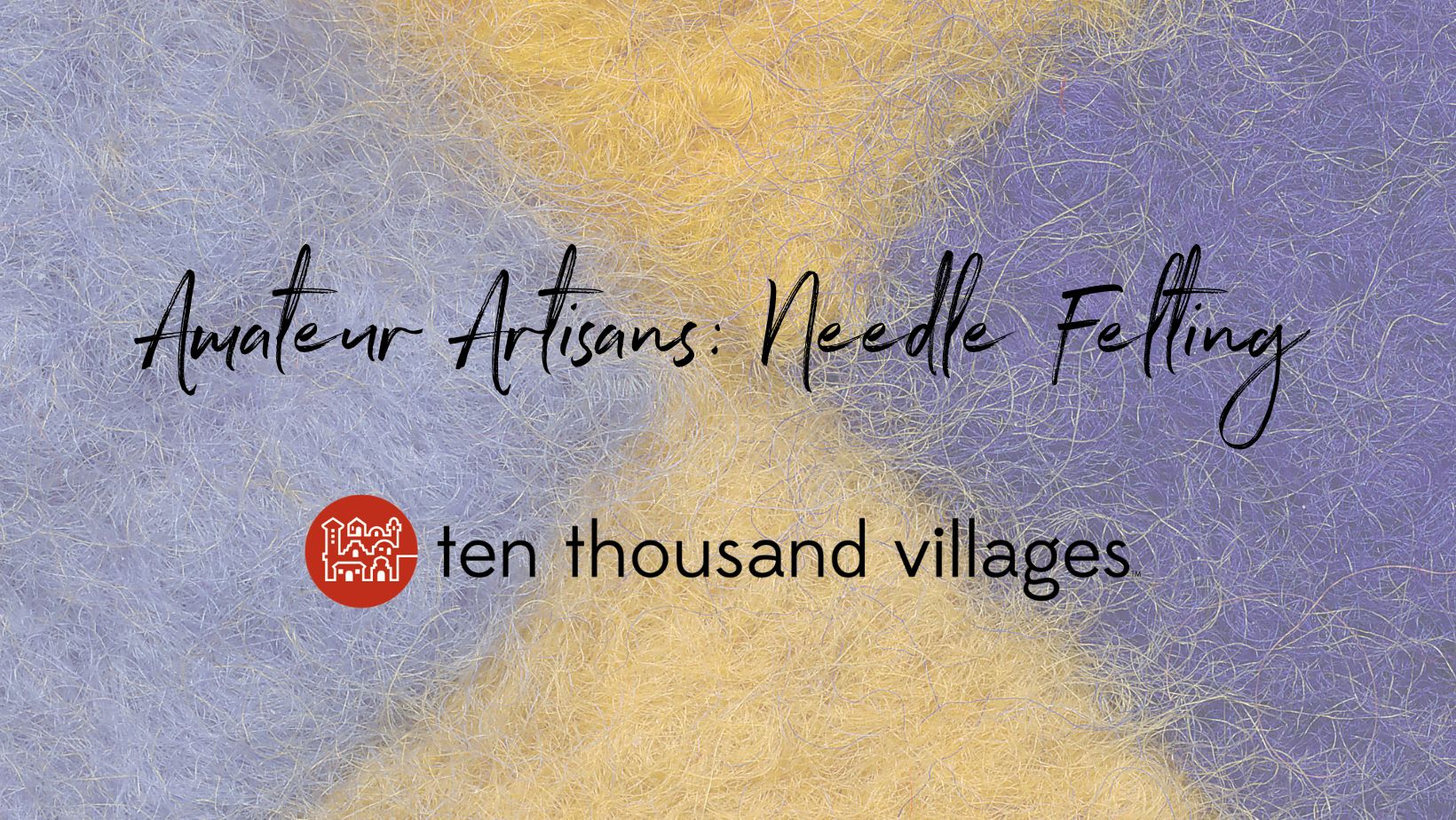The image appears to be a flyer or business card featuring a central block of text in a handwritten cursive font. The text reads "Amateur Artisans: Needle Felting," and just below it in lowercase, regular script, it says "10,000 Villages." Adjacent to this text on the left is a small red circle logo with a white outline of houses. The background of the image is divided into four triangles: the top and bottom triangles are a light beige color, and the left and right triangles are shades of blue and purple. This textile-like fabric creates a visually appealing and structured background for the central information. The overall color scheme includes yellow, light blue, dark blue, black, white, and red, giving it a vibrant yet cohesive look.